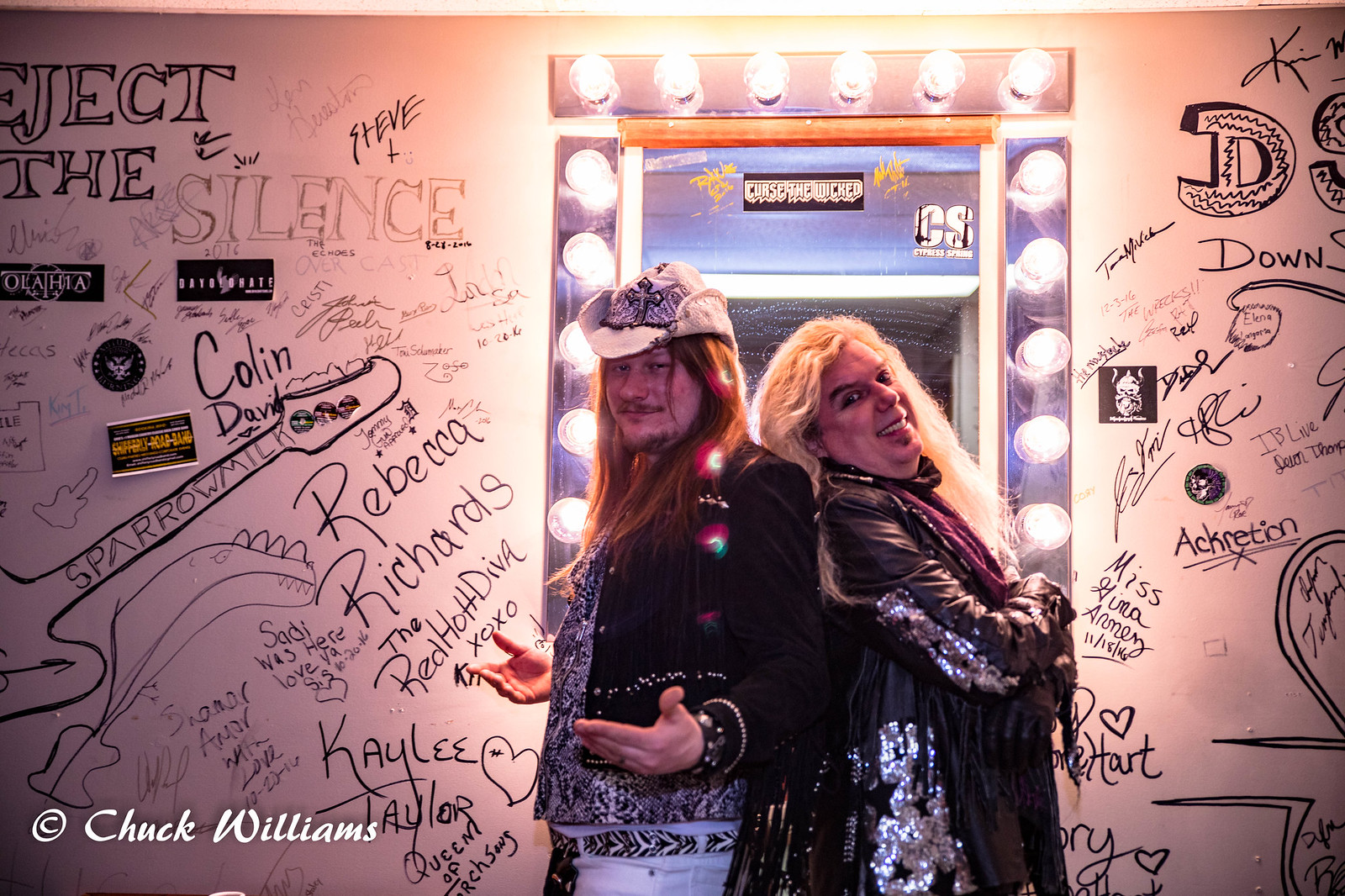In the image, two men are posing with their backs to each other, each displaying distinct body language. The man on the left, adorned with a cowboy hat featuring a cross, has his hands lifted with palms up and appears to be gazing at a calendar. He exudes a contemplative aura. Contrastingly, the man on the right tilts his head back, gazing directly at the camera with his arms crossed in front of him, portraying a confident demeanor. Both men have very long hair that adds to their striking presence.

Behind them is a mirror framed with large light bulbs, contributing to a theatrical ambiance. The backdrop features a white wall covered in an array of signatures, drawings, and graffiti, suggesting a lively and creative environment. On the left side of the wall, notable signatures include "Eject the Silence" in black marker, "Colin David," "Rebecca Richards," "The Red Hot Diva, XOXO," and "Kaylee Taylor," with a detailed drawing of a guitar labeled "Sparrow Milk." The right side of the wall showcases names such as "Ackerton" (possibly "Accretion"), "IB Live," and "Miss Puma" in cursive, with additional illustrations including a dragon and hearts.

In the bottom left corner of the image, a watermark reads "© Chuck Williams," indicating the photographer or artist.